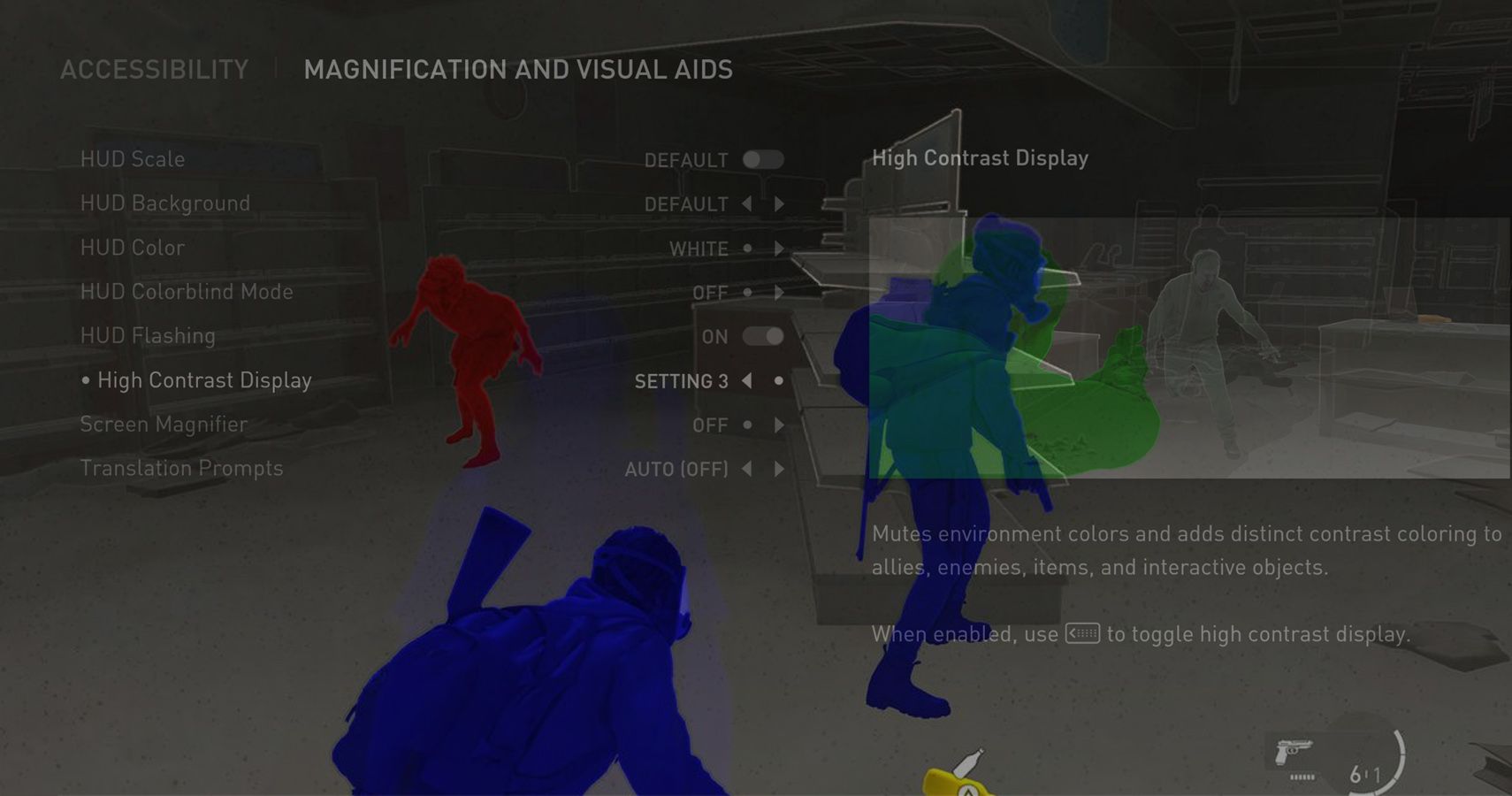This image depicts a dark, game-like screen with a predominantly blackish-gray background. At the top, white text reads "Accessibility, Magnification, and Visual Aids." Below this, various HUD (Heads-Up Display) settings are listed vertically, including "HUD scale: Default," "HUD background: Default," "HUD color: White," "HUD color blind mode: Off," and "High Contrast Display: Setting 3." 

In the background, there is a grayscale room scene with three distinct figures: two blue-glowing soldiers holding guns, and a red-glowing figure crouching to the left whom may represent an enemy or distinctive character. The blue soldiers are dressed in military uniforms and protective gear, indicating readiness for combat. The red figure, possibly a monster or a significant enemy, adds tension.

On the right side of the image, a paragraph explains the functionality of the high contrast mode: "Mutes environment colors and adds distinct contrast coloring to allies, enemies, items, and interactive objects. When enabled, use the arrow to toggle high contrast display."

Overall, the screen is rich with accessibility features, emphasizing contrasting visual elements to aid different players.